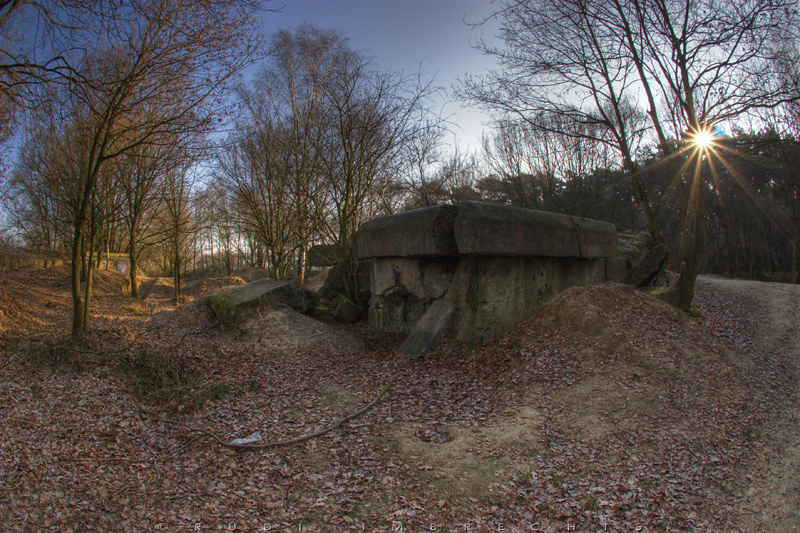The image depicts a serene, late fall landscape under a predominantly blue sky, tinged with hues suggesting either a sunrise or sunset on the right side. The sky transitions into a backdrop of leafless trees, occasionally specked with a few remaining leaves. The ground below is carpeted in a dense layer of brown, fallen leaves, interspersed with bare patches of dirt. Dominating the center of the scene, a stone formation, possibly man-made, stands as a focal point. This stone structure appears to be a rectangular platform with a rounded top edge and an additional layer on top, surrounded by large boulders at varying levels. The exact purpose of this stone formation remains unclear.